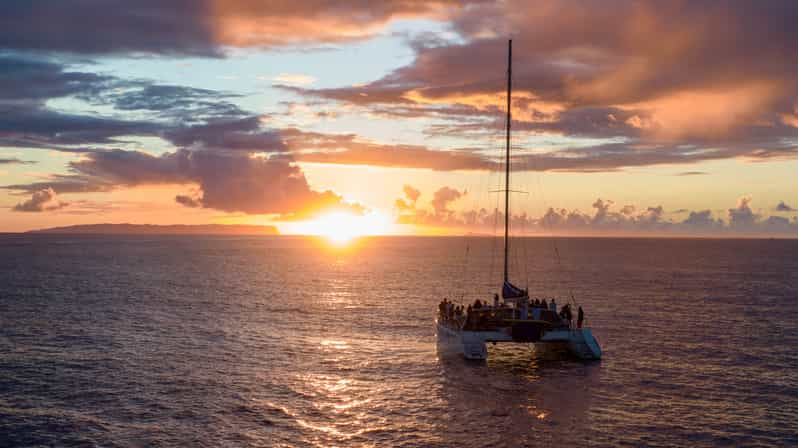The image captures a breathtaking sunset over the ocean. The glowing sun, positioned in the center just above the horizon, bathes the scene in a vibrant yellow-orange light, creating a stunning transition from dark clouds near the horizon to a light blue sky with scattered gray and purple clouds higher up. On the ocean's surface, the water shimmers with the sun's reflection forming a gleaming line down the center. Toward the bottom right of the picture, a white catamaran is filled with silhouettes of numerous people, estimated around 20. The boat has no visible sail, but its tall mast, accompanied by several guy wires, stands out against the sky. The catamaran's unique structure allows you to see water through the space between its two hulls. In the background, there is a hint of land with a significant cliff drop-off, adding depth and context to the expansive sea. The overall composition beautifully balances the bright sunset, the serene sea, and the lively boat teeming with people.